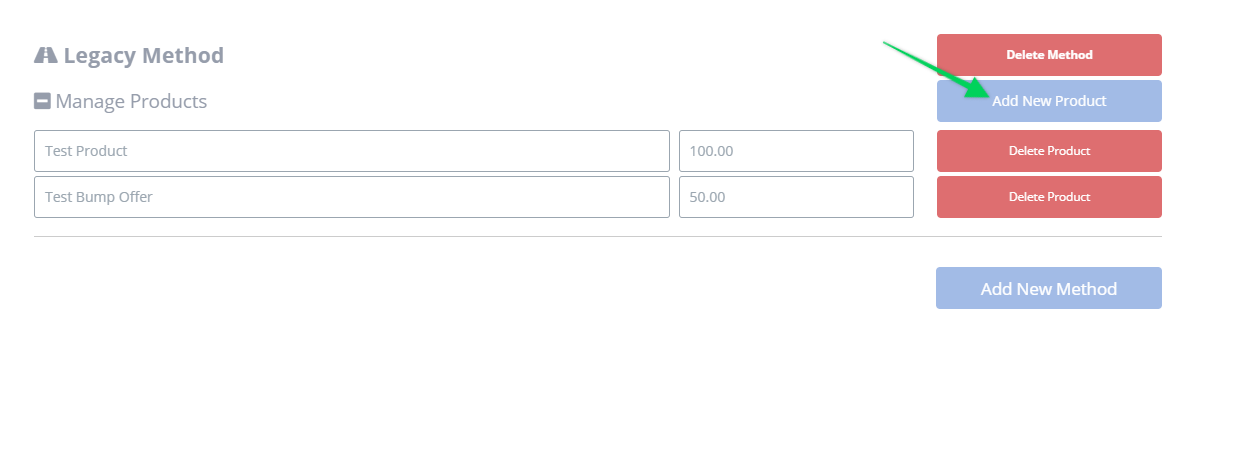The image depicts a user interface for managing products within a legacy system. The UI features various sections and fields, prominently including "Legacy Method," "Manage Products," and two specific fields titled "Test Products" and "Test Bump Offer." Adjacent to "Test Products" is the figure "$100.00," and next to "Test Bump Offer" is "$50.00." To the right, there are several actionable options including "Delete Method," "Add New Product," and twice-listed "Delete Product." An arrow is pointing towards the "Add New Product" box, indicating an emphasis on this area. At the bottom, there is another box titled "Add New Products," hinting at additional product management functionalities. The color scheme of the interface consists of red, white, and gray, primarily used for the text and various elements.